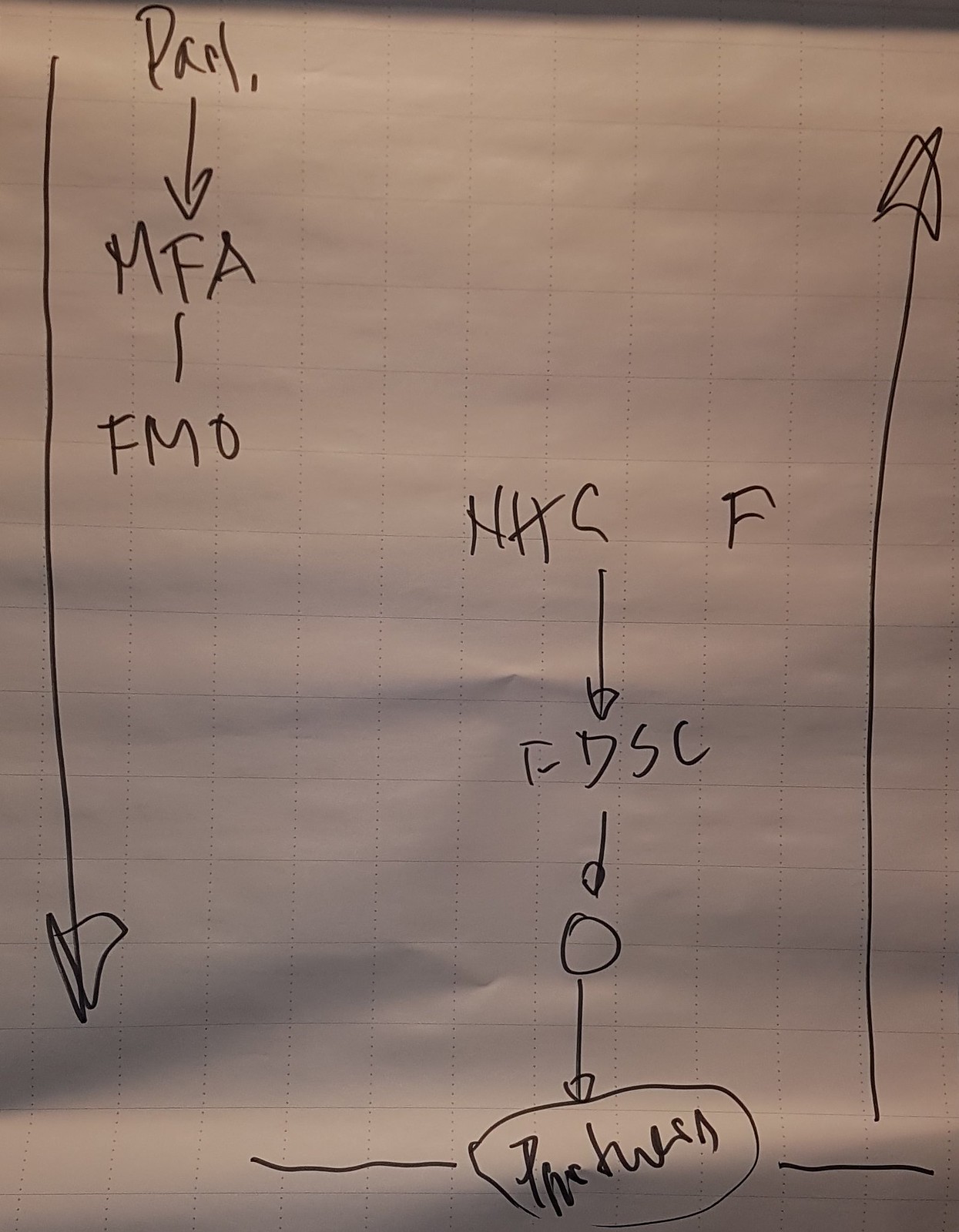The image captures a white sheet of perforated paper, with multiple interconnected arrows and various text annotations suggesting an unknown process or formula. The rightmost arrow, positioned vertically, points upward from near the bottom to nearly the top of the image. On the left side, there is another vertical arrow that points downward, starting from the top and extending almost to the bottom.

In the top left corner, just beside the downward-pointing arrow, there's text that reads "PARL," followed by a small downward arrow, then "MFA." Beneath this is another line of text that says "FML." Near the bottom right corner, to the left of the area, a circled text can be observed, although it is faint and appears to spell "PNCHLSA."

Two horizontal lines, one on the left and one on the right side of the image, are present without any accompanying text. Around the middle section of the upward-pointing arrow on the right, there is text that seems to begin with "NHC," followed by a space and the letter "F." Further down, a small downward arrow directs to text that reads "FDSC," which is followed by another small arrow. This points to a circled area that again connects to the earlier mentioned circled text.

All these annotations and graphic elements are laid out on a white perforated sheet, containing approximately 20 intact perforations, forming a grid of small squares. The text is in black, contrasting against the white background, making the details distinct.